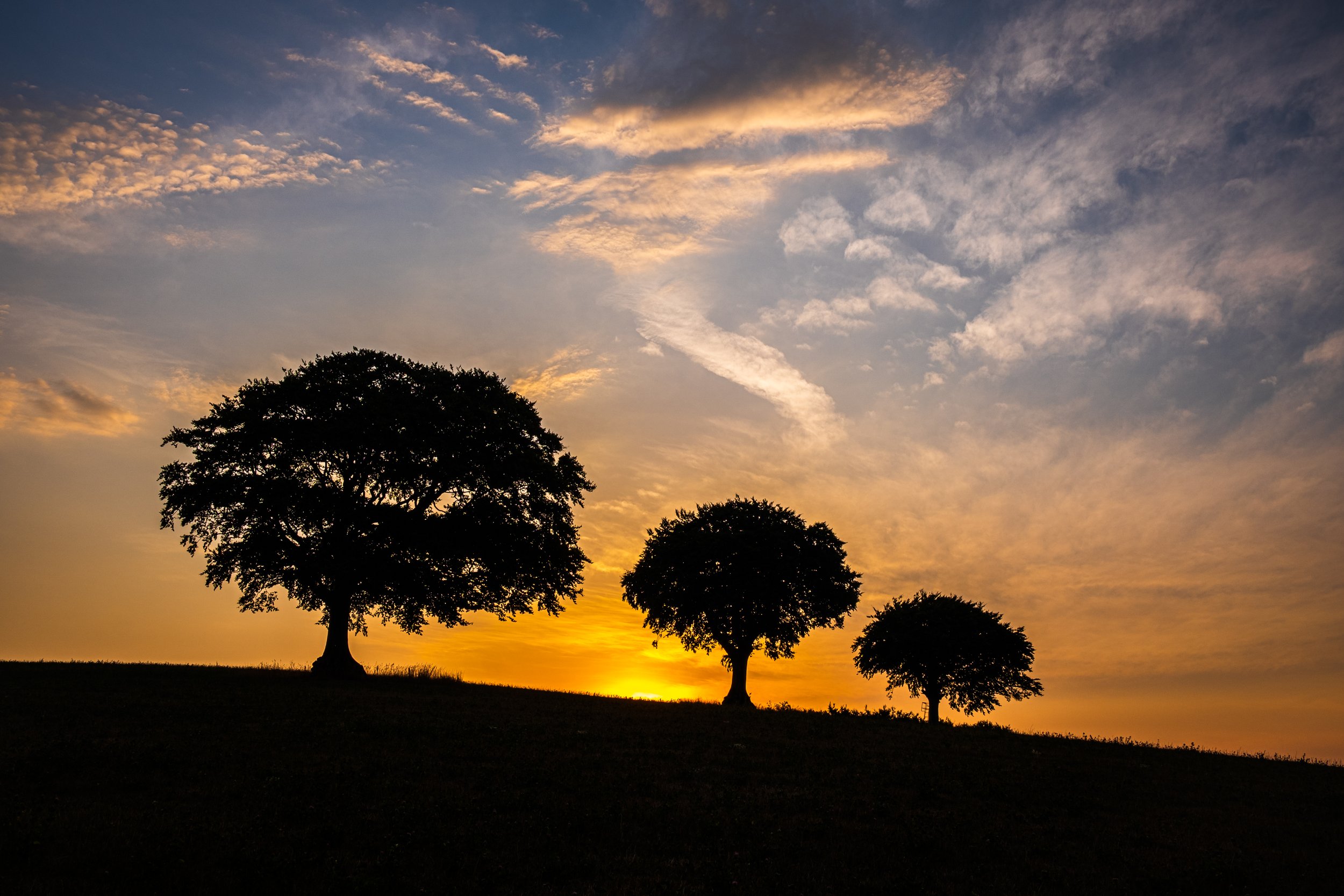This captivating image features a stunning, dramatic sky with deep shades of blue and gray, interspersed with delicate streaks of pink and purple. Wispy, string-like clouds stretch across the horizon, highlighted by a striking, prominent white dash. Beneath this vivid sky, the sun sets with a radiant display of golden and purplish hues, casting a warm glow over the landscape. In the foreground, a dark, rolling hill provides a stark contrast to the vibrant sunset. Three majestic trees, each progressively larger and adorned with lush green foliage, stand prominently on the hill, their rounded canopies adding a touch of natural beauty to this serene and enchanting scene.